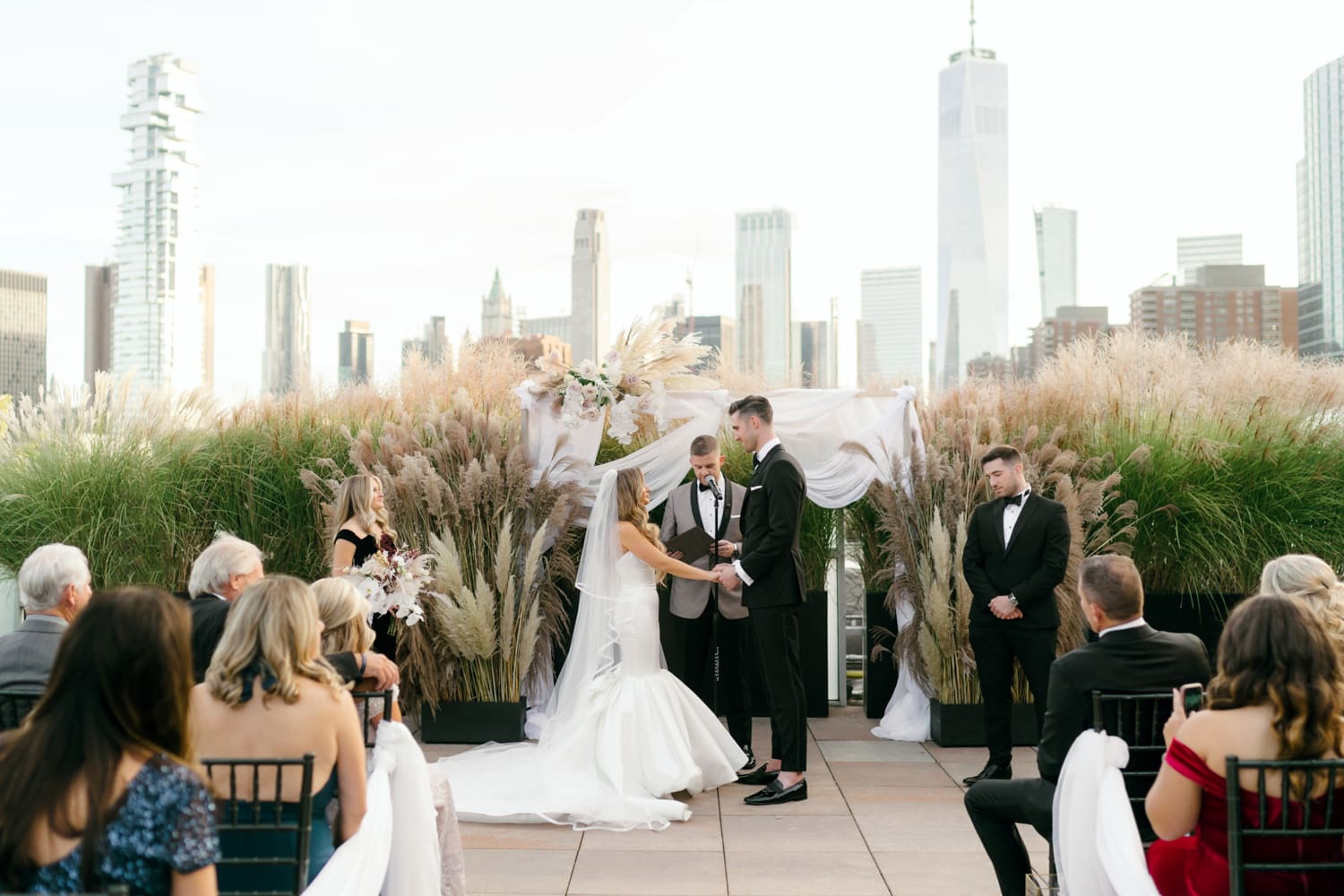In this richly detailed photograph of an outdoor wedding, we see a rooftop ceremony set against a cityscape backdrop with numerous tall buildings in view. In the foreground, guests are seated with their backs to the camera, attentively watching the event. Center stage, a bride with long, blonde, wavy hair is adorned in a white fit-and-flare dress with a fishtail bottom and a flowing veil. She stands on the right, holding hands with the groom, who is dressed in a dark suit and tie, noticeably without socks and with short, dark hair.

Flanking the couple are the bridal party members: to the groom's right stands the best man in a similar tuxedo, while to the bride's left, the maid of honor is elegantly dressed in a dark-colored gown and holding a bouquet. Directly behind the bride and groom, the officiant, wearing a light brown suit with a darker collar, looks down at a book.

The setting features lush decorations, including an elaborate floral archway draped with white satin behind the officiant. Surrounding the couple are tall cattail grasses with green stems and puffy cream-colored tops, as well as a prominent station of pampas grass to the left. This meticulously orchestrated scene captures the intimate and elegant atmosphere of the wedding ceremony.